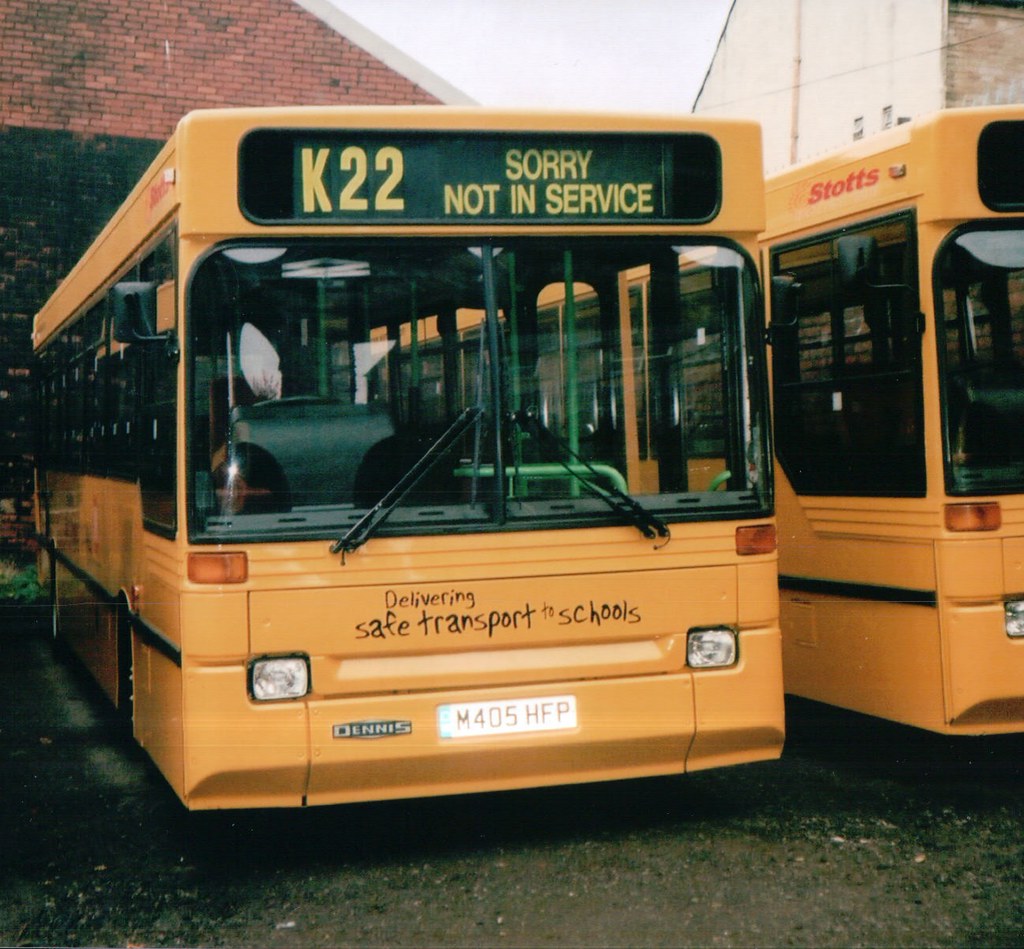In the photograph, a prominently yellow school bus is parked with its clear front windows reflecting the surroundings. The digital display at the top of the bus reads "K-2-2 sorry not in service." Directly beneath the windows, the front of the bus bears the phrase, "Delivering safe transport to schools." Near the bottom corner, the bus features a "Dennis" logo. The front license plate and headlights are also visible, neatly integrated into the design. Next to it, on the right, the partial side view of a similarly styled second bus can be seen. This second bus showcases a red "Stotz" logo on its upper section. Despite being cut off partially, the distinct similarities in design confirm it as the same model.